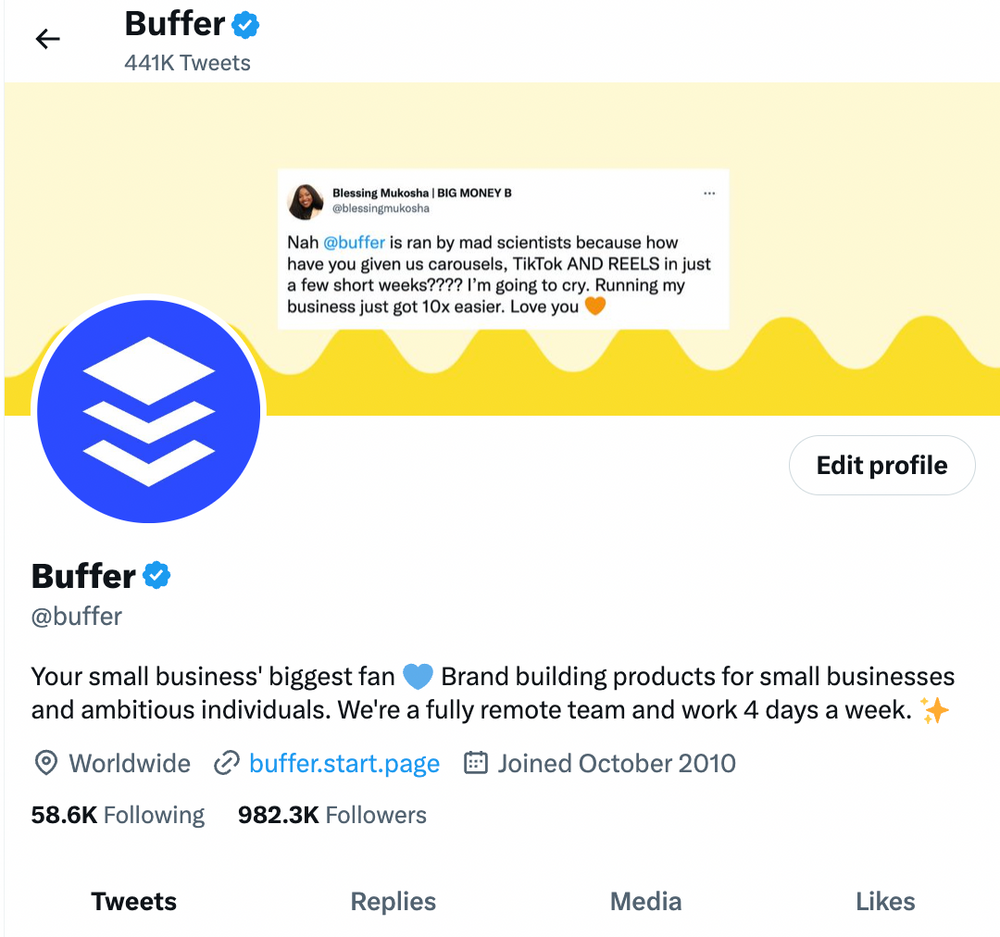The image showcases the Twitter profile page of Buffer, a verified account. At the top, the bold word "Buffer" is displayed alongside a blue verified badge. Below, in gray text, "441,000 Tweets" indicates the account's tweet count.

The main highlight is a light pink rectangular graphic with a gold, ocean wave design at the bottom. Inside this box, a post by a Twitter user, Blessing Mukosha, known as "Big Money B," is displayed in a white box. The post reads: "Nah, Buffer is ran by mad scientists because how have you given us carousels, TikTok, and Reels in just a few short weeks? I'm going to cry. Running my business just got 10 times easier. Love you," followed by an orange heart emoji.

At the bottom-left of the graphic, the Buffer logo partially overlaps the white background. The logo consists of a bright blue circle with a white border and an accordion-like design in blue and white.

To the right of the pink graphic, there is a white button with a gray border that reads "Edit Profile" in black text.

Further down, the word "Buffer" appears again in bold black print with the verified badge. Beneath, the bio section reveals: "Your small business's biggest fan 💙 Brand building products for small businesses and ambitious individuals. We're a fully remote team and work four days a week ✨." The location, "Worldwide," and "Joined October 2010" are shown in gray.

Buffer follows 58.6 thousand accounts and is followed by 982.3 thousand users. The navigation bar at the bottom offers tabs for "Tweets," "Replies," "Media," and "Likes."